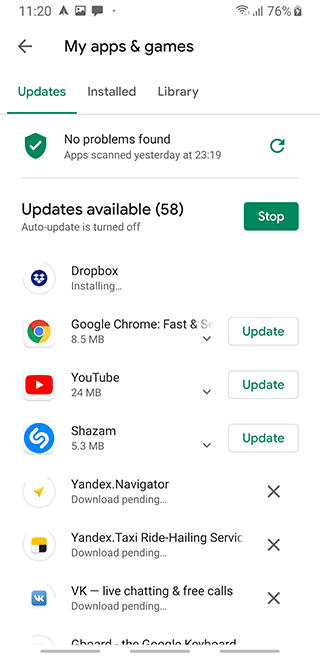The image captures a smartphone screen displaying the updates interface for applications. Positioned in the top left corner is the time: "11:20." The top right corner features various status icons, including those for internet connection, cellular signal, a charging battery marked at "76%," and the time.

Centered below these icons is a header titled "My Apps and Games," flanked by three tabs labeled "Updates," "Installed," and "Library," with the "Updates" tab currently selected. Directly below this, a shield or badge icon with a white arrow inside it signifies system status, accompanied by text stating: "No Problems Found. Apps scanned yesterday at 23:19."

Continuing downward, it indicates there are "Updates Available: 58," and notes that "Auto-update is turned off," with a prominent green button labeled "Stop" in the middle. Below this section, a white circle icon denotes that "Dropbox" is currently installing.

Further down, the display lists app details one by one:
- A white square with the Google logo, labeled "Google Chrome, Fast (8.5 MB)," alongside an "Update" option with a white background.
- A square featuring the YouTube logo, captioned "YouTube (24 MB)," with an adjacent white "Update" button.
- The Shazam icon with the label "Shazam" next to a white "Update" button.
- The Yandex Navigator icon, accompanied by the note "Download Pending."
- The Yandex.Taxi icon, stating "Yandex.Taxi Ride Hailing Service, Download Pending."
- The VK Live icon reading "VK Live, Chatting and Free Calls, Download Pending."

This detailed snapshot provides a comprehensive view of the app updates screen, ensuring users can readily identify the status of their applications and available updates.